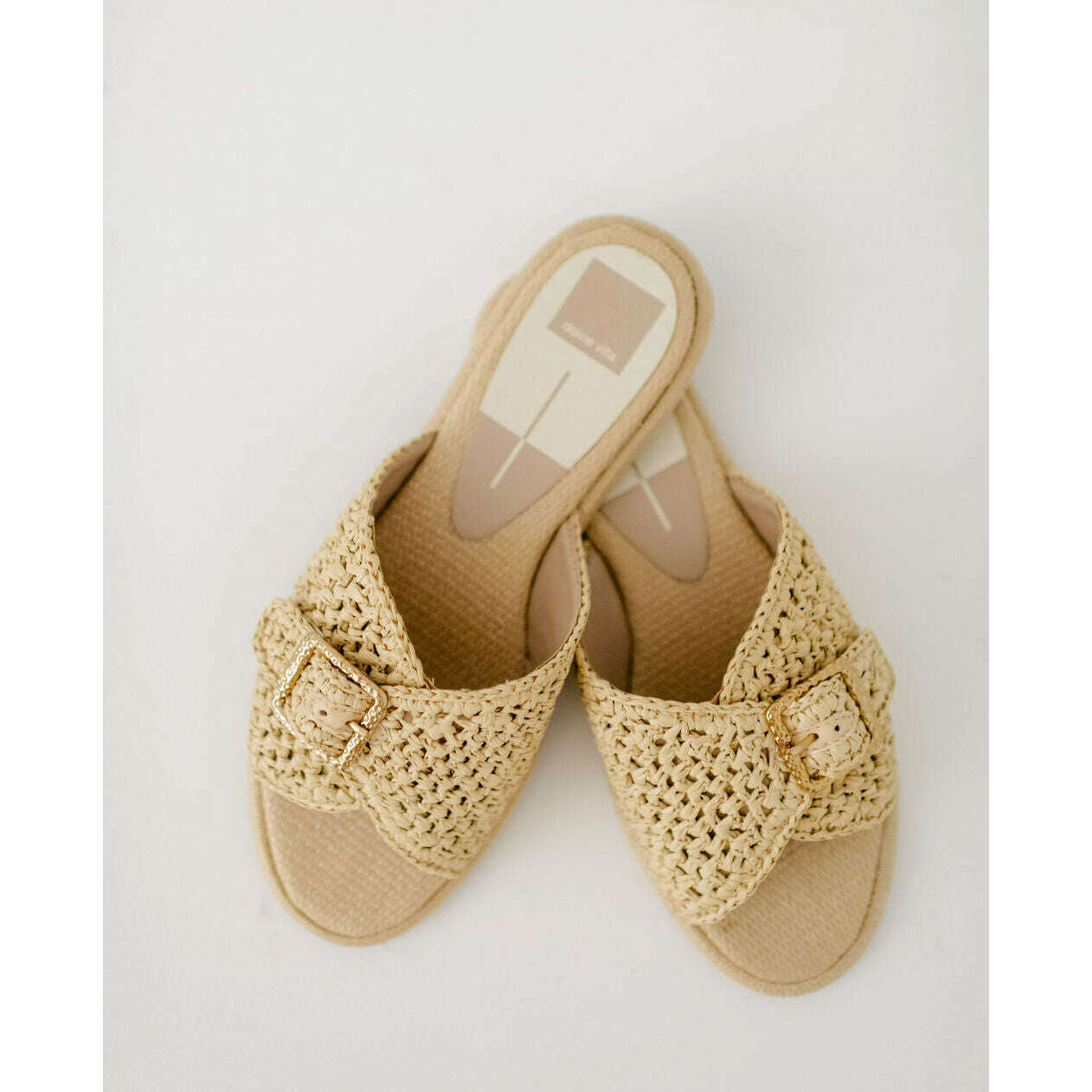This is a detailed close-up photograph of a pair of stylish, open-toe sandals captured from above. The sandals rest on a plain, off-white, beige background with one shoe positioned over the other. The footwear showcases a distinct design with a combination of tan and cream colors. The footbed where the feet would rest is tan, while the crisscrossing, woven upper part, reminiscent of a jute or wicker fabric, is cream, featuring breathable, crocheted-like holes.

A prominent feature of these sandals is the oval shape at the heel area, split into light and dark beige tones. A square, also located towards the front with illegible white writing, suggests branding elements not clearly visible in the image. The sandals are secured with a hammered gold buckle, positioned on the fourth hole, enhancing their chic appeal. The base of the shoes appears cushioned, providing added comfort and slight arch support.

Overall, these sandals, potentially from the "Dalla Vita" brand, blend practical comfort with elegant design, making them a fashionable choice for various occasions.